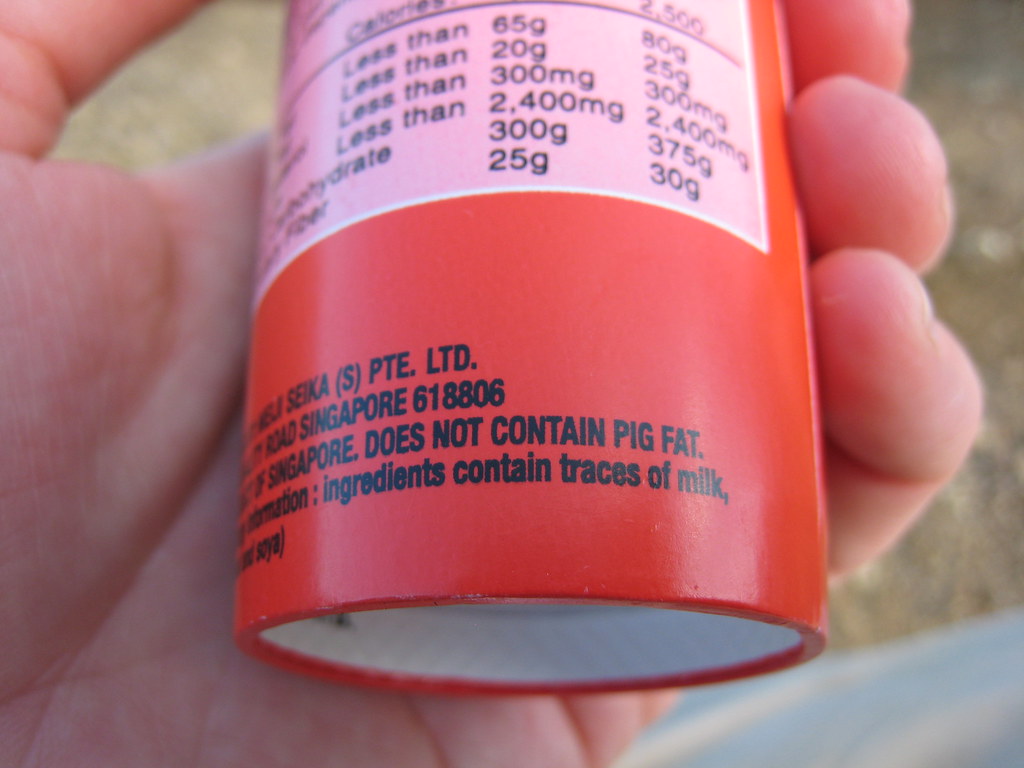The photograph depicts the close-up of a white male hand holding a small, cylindrical, orange container in the palm of his hand. The container, about the size of a standard retail single-serving bottle, features a nutritional content label on a light pink background with black letters. The visible part of this label lists calories and several values in grams and milligrams, such as 65g, 80g, 20g, 25g, 300mg, and 2400mg. The contents of the label are partly obscured. 

Below the nutritional information, the label indicates that the product does not contain pig fat and might contain traces of milk. Manufacturer details are found at the bottom in black lettering, stating "CKSPTE.LTD" and "Singapore." The hand holding the container prominently displays the palm, pinky finger, ring finger, and part of the middle finger, while the thumb is partially visible.